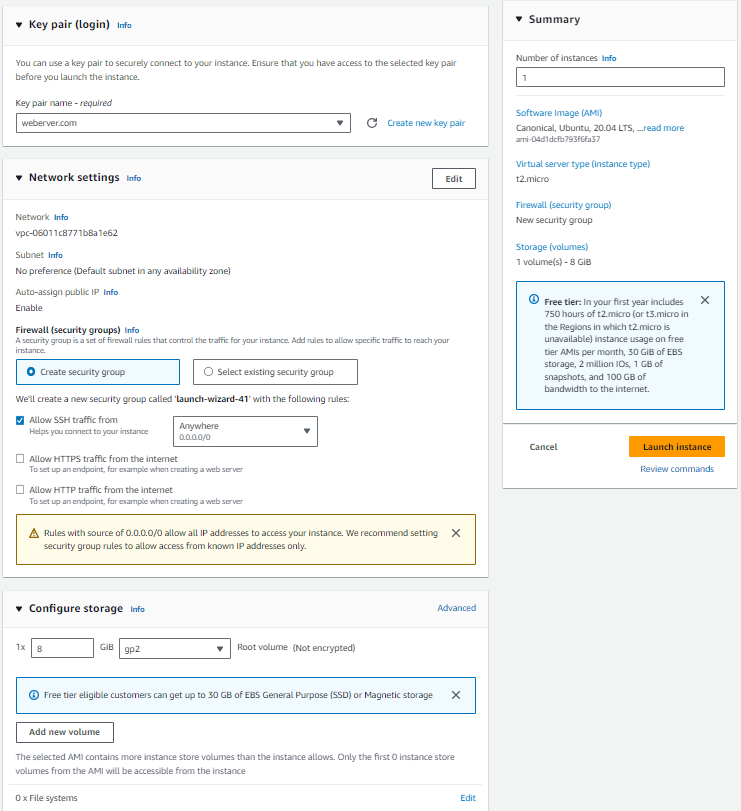Title: Screenshot of Key Pair Login Interface for Secure Authentication

Description:
At the top of the screenshot, "Key Pair Login" is prominently displayed in bold black text. Below this title, "Info" is written in blue, indicating a section containing additional information. Adjacent to this, a downward-pointing arrow directs the user to further details. This section informs the user that a key pair can be utilized to enhance website security. 

Continuing downward, another arrow points towards a 'Replay' button, followed by an option to "Create a New Key Pair." Below this, the interface includes a "Network Settings" section, with an additional downward-pointing arrow leading to it. 

In the "Network Settings" area, there is a yellow box and a blue box, each with specific configuration settings. Next to these boxes, a small caption states "Configure Settings," suggesting that users can add or modify information within these settings.

To the right side of the screenshot, a blue-highlighted box provides a summary of all the elements described on the left side of the interface, enabling users to quickly review key information and ensure accuracy in their configurations.